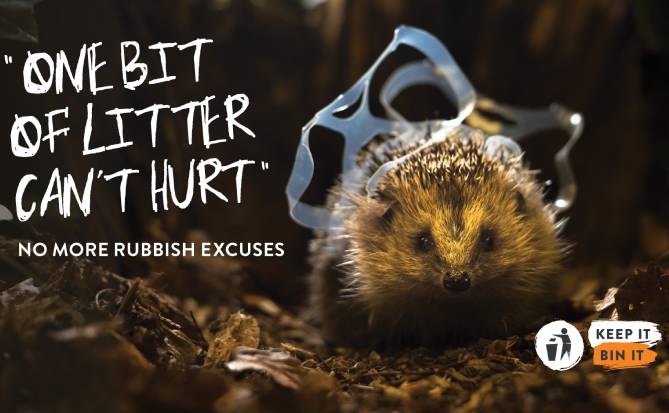The photograph captures a poignant scene set against a dark forest floor scattered with dirt and leaves. In the lower right corner, a small, furry animal with brown fur—resembling a hedgehog or porcupine—is ensnared by a plastic six-pack ring, highlighting the distress caused by environmental negligence. On the upper left, text in a sketchy, handwritten style reads, "One bit of litter can hurt," with a somber tone echoed in the smaller font below: "No more rubbish excuses." The image's impact is further enhanced by a public service announcement feel, emphasized by a circular logo in the lower right showing a figure disposing of trash. Beside the logo, a white and orange swatch declares a final plea: "Keep it, bin it."